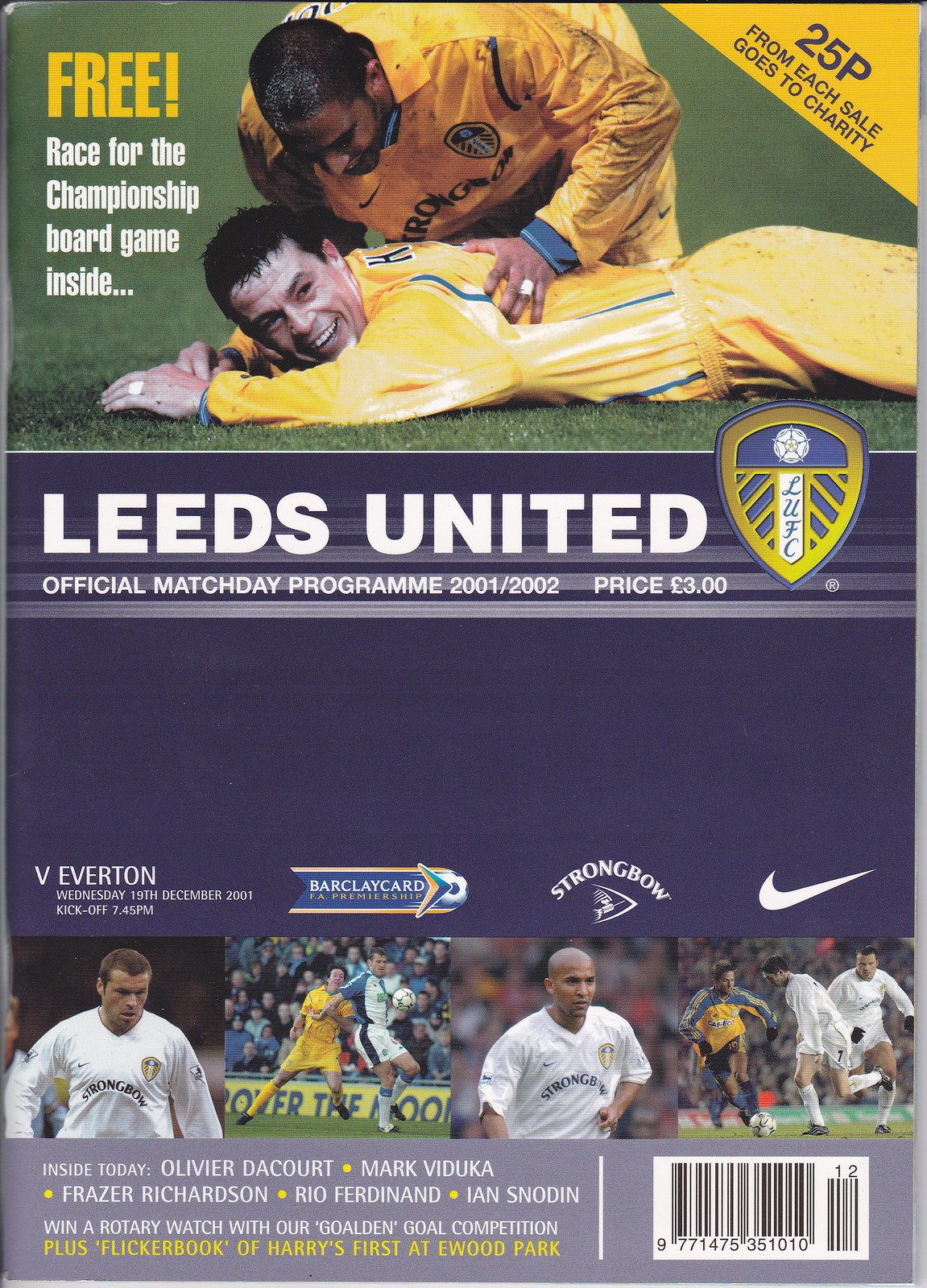This is the cover of the Leeds United Official Match Day Program for the 2001-2002 season, priced at £3. The top third features a green background with a photograph of two soccer players in yellow uniforms with blue stripes; one player is lying on his stomach on the grass, while the other leans over him, possibly massaging his shoulder. On the left side, in yellow text, it says "FREE!," followed by "Race for the Championship Board Game Inside" in white text. In the top right corner, a yellow triangle with black text reads, "25p from each sale goes to charity." The bottom two-thirds of the cover has a blue background with multiple lines of text and photographs. The central area includes the title, "Leeds United Official Match Day Program 2001-2002," along with the LUFC shield logo. Below, it mentions the fixture "V Everton," accompanied by various company logos, including Nike. There are four photos of soccer players like Olivier Dacourt, Mark Viduka, Frazer Richardson, Rio Ferdinand, and Ian Snodin, along with additional information about the included content. A barcode is located in the bottom right corner.